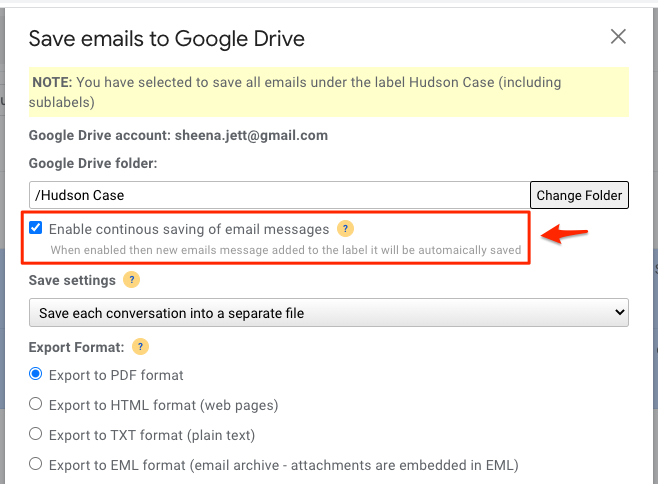A highly detailed and organized screenshot captures a pop-up interface for saving emails to Google Drive. The upper right-hand corner features a clickable 'X' for closing the window. At the top of the pop-up, bold text reads, "Save emails to Google Drive." Beneath this, inside a prominent yellow rectangle, there's a notice: "Note: You have selected to save all emails under the label Hudson Case, including sub-labels." 

Further down, the Google Drive account is specified as "SheenaJett@gmail.com," and the targeted Google Drive folder is named "Hudson Case." A red triangle beneath this warns, "Enable continuous saving of email messages." Adjacent to this warning is a checkbox that is checked, signifying that continuous saving is active. A red arrow points clearly to this enabled checkbox.

Below these elements, there is a "Save Settings" button. A drop-down menu below this button indicates the format preference: "Save each conversation into a separate file" is selected. Following this option, an "Export Format" section offers several choices for file format. The radio button next to "Export to PDF format" is selected, while the other options – "Export to HTML format," "Export to text format," and "Export to email format" – remain unselected.